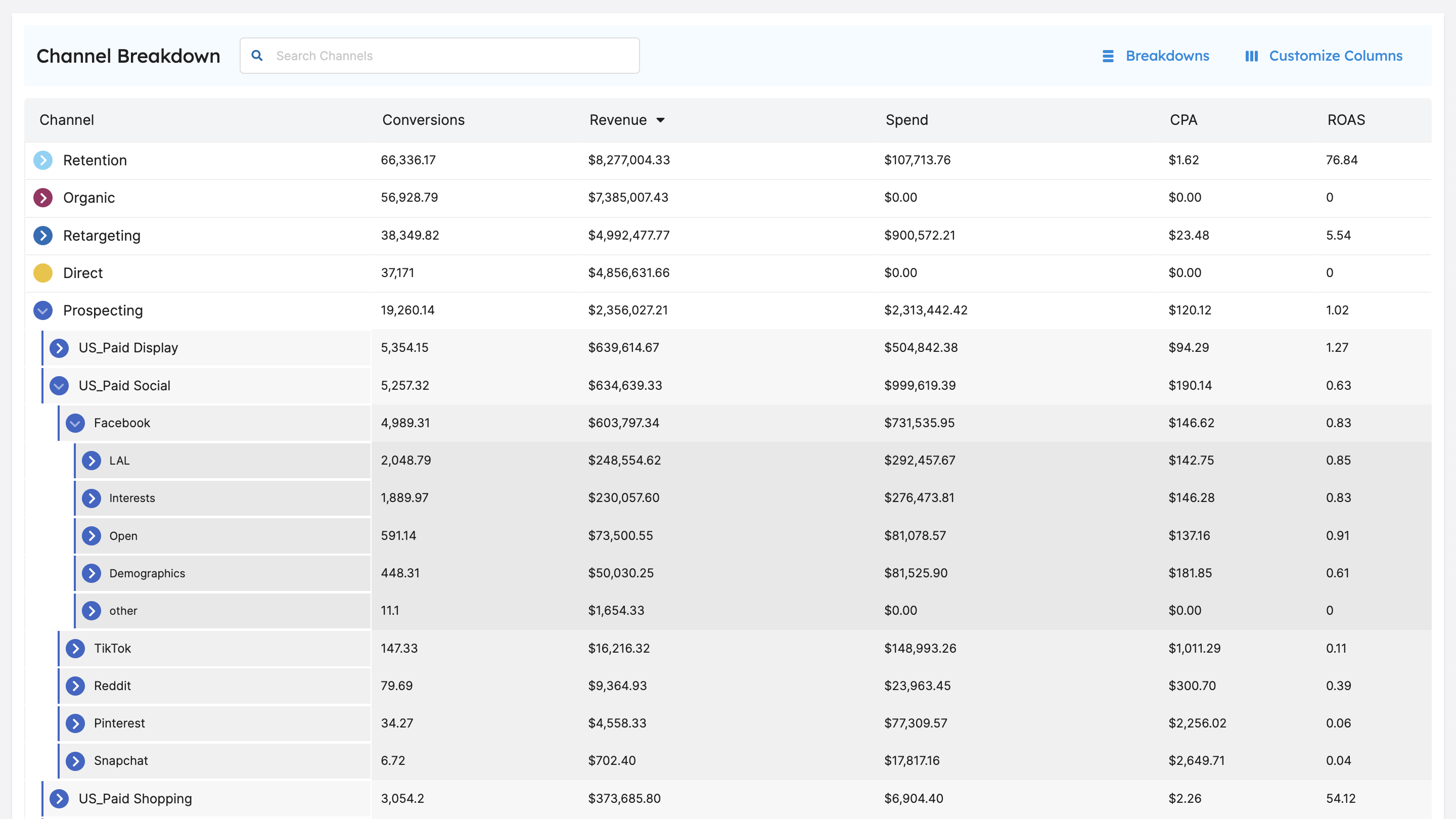The image displays a detailed screen titled "Channel Breakdown" located at the top left corner. Directly beneath the title is a search box equipped with a magnifying glass icon for channel search functionality. 

To the right of the screen, blue text headlines capture attention: "Breakdowns" and "Customize Columns." Below, the columns are systematically arranged into sections labeled Channel, Conversions, Revenue, Spend, CPA, and ROAS.

At the top of the list is the "Retention" channel, reporting the following metrics: 
- Conversions: 66,033.617 
- Revenue: $8,277,004.33 
- Spend: $107,713.76 
- CPA: $1.62 
- ROAS: 76.84

Following "Retention" is the "Organic" channel accompanied by similar metrics. Other channels listed are "Retargeting," "Direct," and "Prospecting." The "Prospecting" category is expanded, revealing several sub-categories:
- US Paid Display
- US Paid Social
  - Facebook (with a down arrow indicating further sub-categories like LAL, Interest, Open, Graphics, Other)
  - TikTok
  - Reddit
  - Pinterest
  - Snapchat
- US Paid Shopping

Each sub-category includes additional specific metrics, all organized to offer a comprehensive breakdown of channel performance.